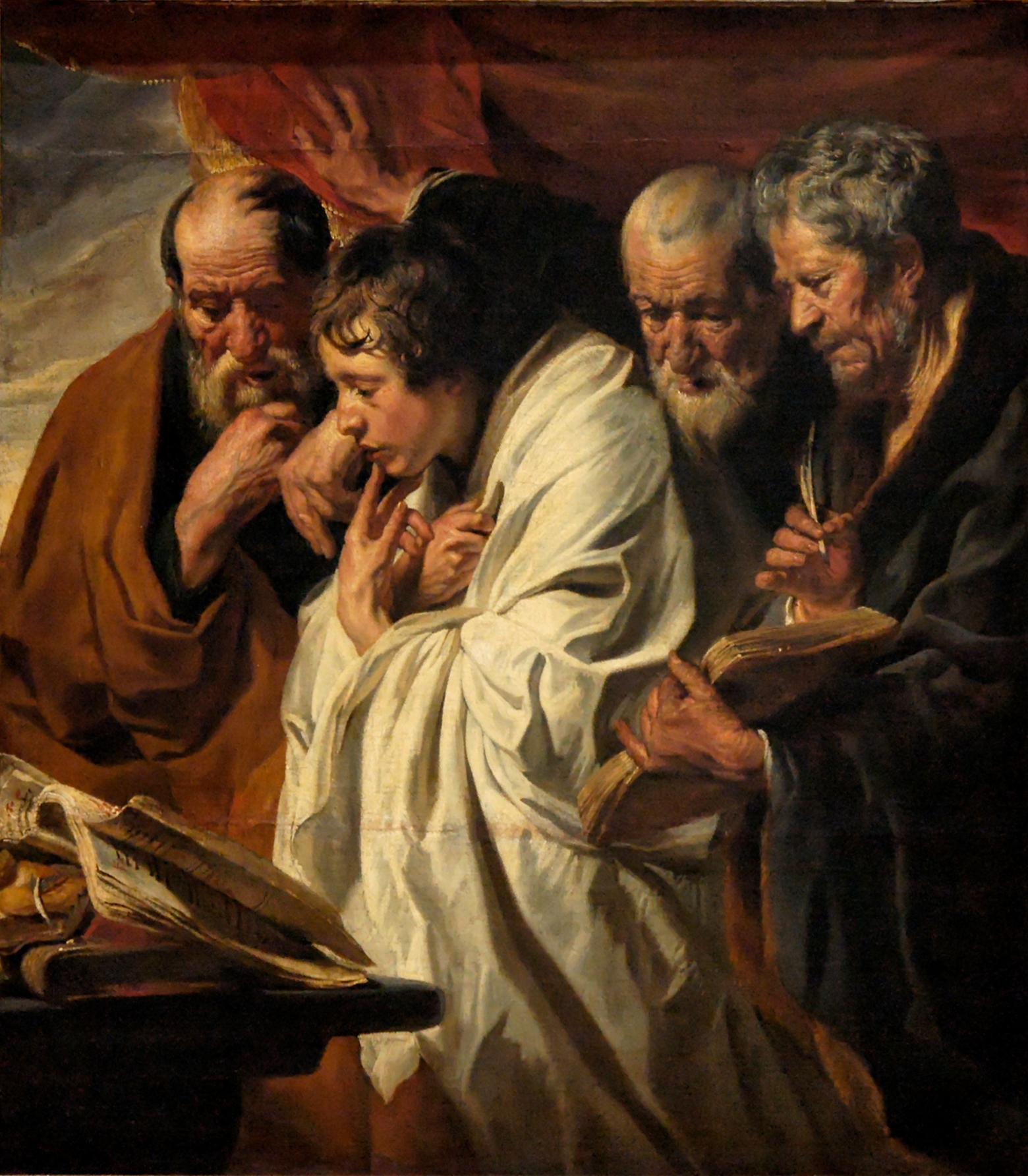The image is a detailed, old-style painting that depicts four individuals against a dark reddish background. Three of the figures are older men, and one is a young boy. The first man on the left side of the painting is wrapped in a brown cloak with thinning dark hair, gray beard, and mustache, appearing to be around 80 years old. Centrally positioned, the young boy with brown hair is covered with a white shroud and has his fingers touching his chin, hands on his chest as if he is cold. Next to the boy, on his right, is an older man with graying black hair and a white beard and mustache, also looking around 80 years old. The fourth figure, another older man with dark gray hair, beard, and mustache, is dressed in a black cloak. He is holding an open book in his left hand and a quill in his right. All of the figures are intently focused on the book, which is placed on a wooden stand, suggesting a scene rich with emotion and concentration, reminiscent of masterful paintings displayed in museums such as the Getty Center.